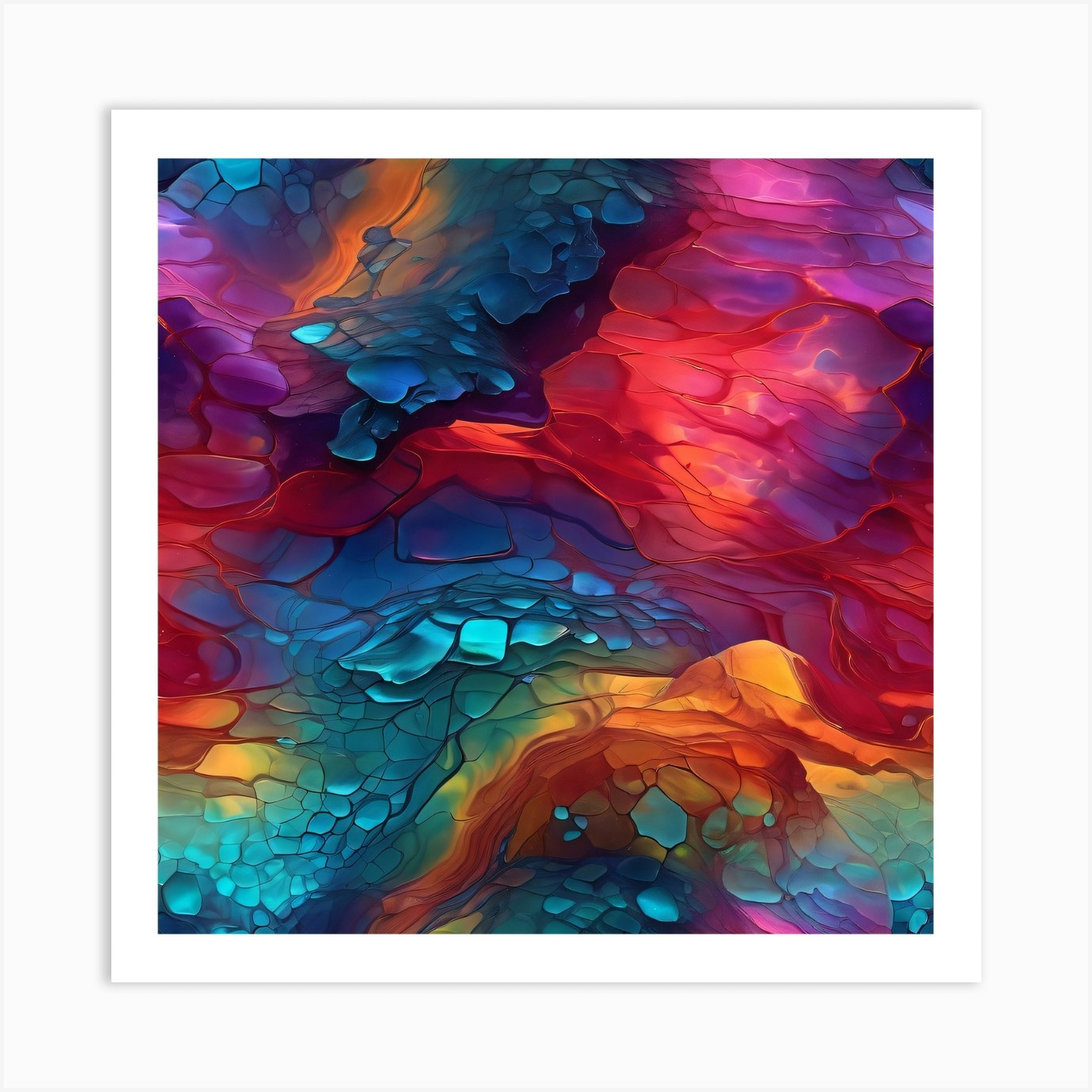The image is a stunning piece of abstract modern art that evokes a sense of vibrant dynamism through its use of brightly colored glass. The overall composition exhibits a kaleidoscopic explosion of hues, including violet, blue, pink, orange, green, yellow, red, and even touches of brown. These colors don't follow the traditional rainbow order but are interspersed in an unpredictable yet harmonious fashion.

The design of the artwork mimics the texture of pebbles and rocks, with sections that give an impression of cloud formations or cliffy, rugged surfaces. Particularly eye-catching are the violet-colored pebbles and the sections with a wave-like, three-dimensional quality. There is a distinct area on the right side that is predominantly pink with purple accents, while another section to the left of the center is mainly blue with hints of green. Light blue rocks intermix with other colors, contributing to the depth and richness of the piece.

This abstract art piece, encased in a white border, draws viewers in with its intricate blend of colors and textures. Its captivating design, reminiscent of scales or fragmented glass, leaves no immediately recognizable objects, allowing for various interpretations and endless visual intrigue.